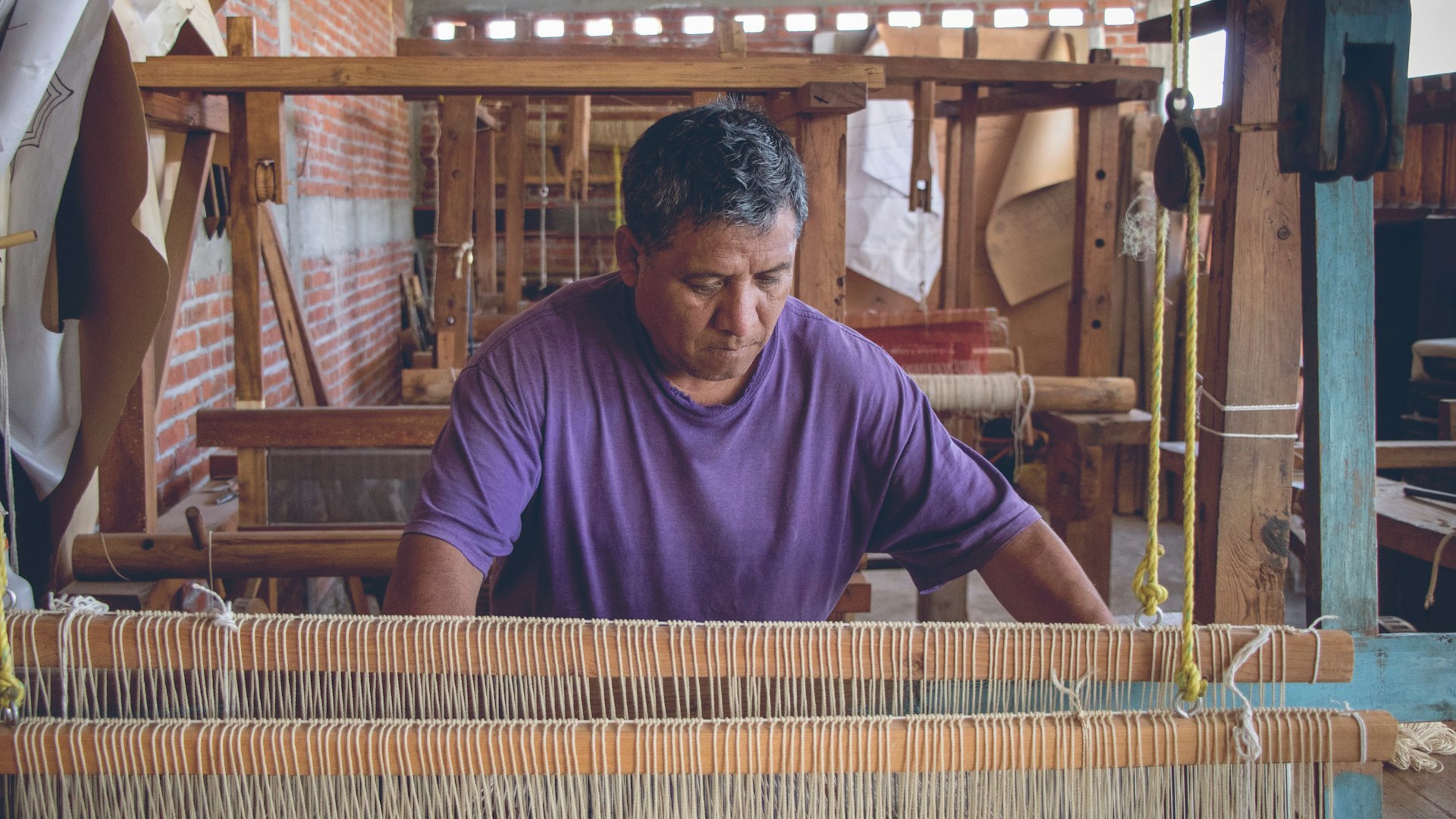In this photograph, we see an older textile worker, likely in his 50s or 60s, intently focused on a traditional fabric or textile piece. He stands at the center of the image, deeply engrossed in his work, reflected in his concentrated expression. The man, who appears to be Asian and has black or gray hair, is dressed in a purple shirt. 

In front of him is a complex wooden device adorned with numerous strings, indicating an intricate and time-consuming task that he is nowhere close to finishing. Surrounding the worker, the setting is a factory with prominent brick walls and machinery positioned both behind him and to his left. A large poster is also visible on the wall to his left. The space is bathed in sunlight streaming in through openings in the wooden structure of the building. The colors in the image include purple, red, blue, white, black, tan, and yellow, adding to the vibrant yet industrious atmosphere of this traditional textile workshop.